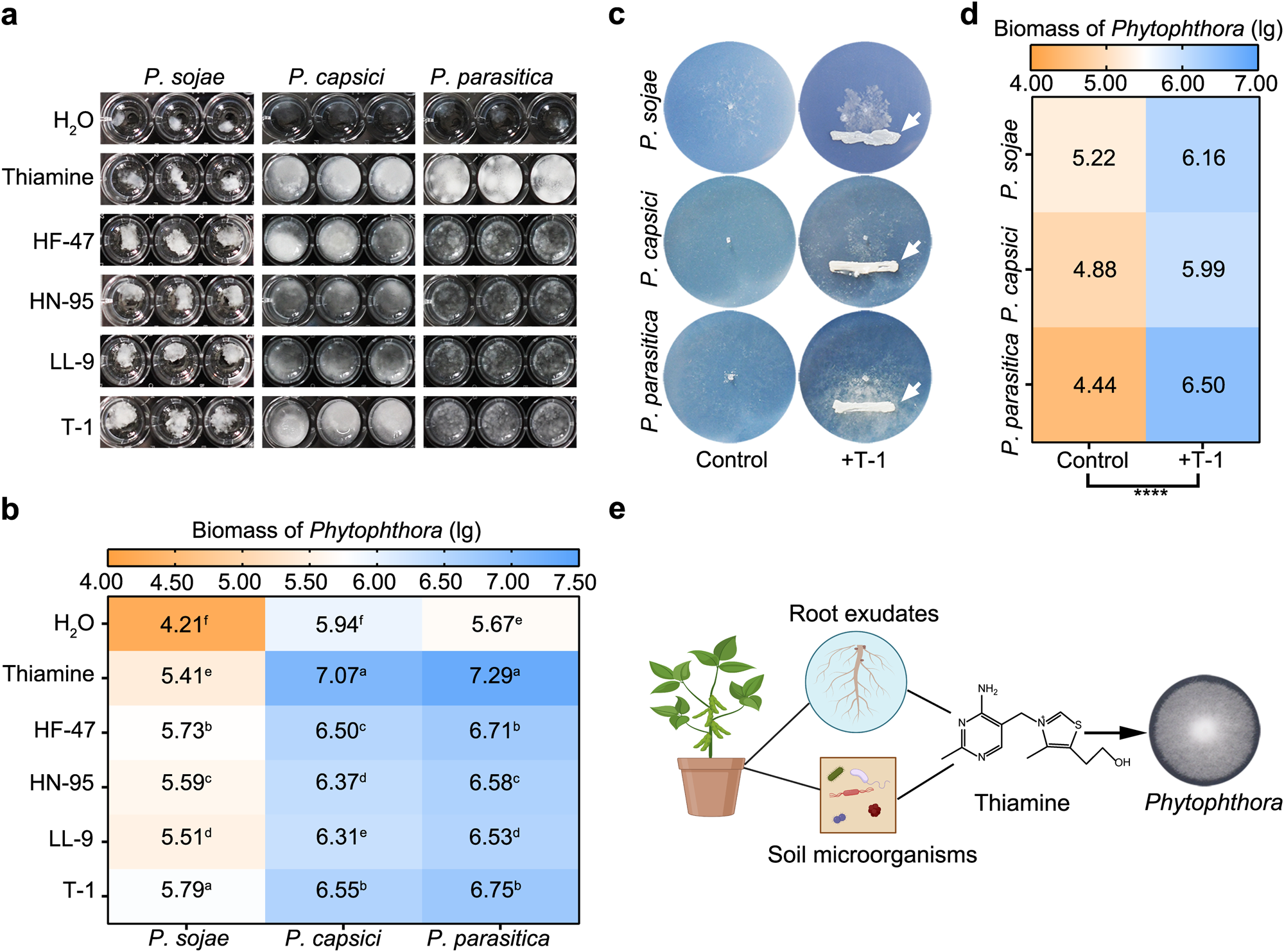The image is a detailed scientific chart focused on plant interactions and chemical processes. In the top left corner, there are black and white photographs labeled P.sojae, P.capsicum, and P.parasitica, showing various organisms growing in agar jars. Below these photographs, a table labeled "biomass of Phytophthora" presents numerical data. To the right, another section with circular photographs displays more images of the same organisms. 

At the center of the chart, a complex diagram illustrates the interactions between a plant in a pot (located at the bottom right), its root exudates, and soil microorganisms. The plant's illustration is connected by arrows to a circle labeled "root exudates" and a square labeled "soil microorganisms," which contains colored depictions of bacteria and other organisms. These elements are linked to a molecule of thiamine, showing chemical structures with N, NH2, and S atoms, which in turn connects to a larger gray circle labeled "Phytophthora."

Overall, the chart moves through sections A to E, incorporating various images, diagrams, and data tables that collectively explore the biochemical interactions between plants, soil microorganisms, and the plant pathogen Phytophthora.